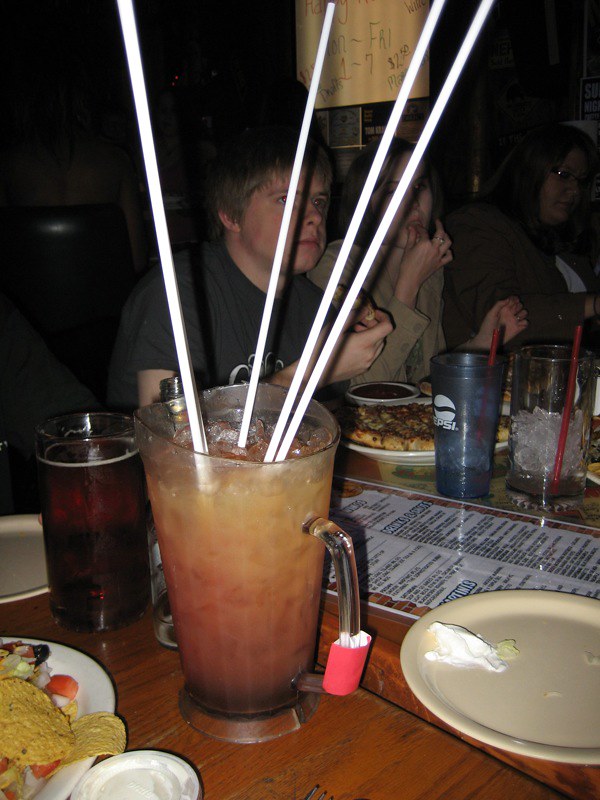This photograph portrays a dimly lit restaurant scene where three individuals are seated around a table, engrossed in their meal. At the center of the table is a large glass pitcher filled with a cloudy, reddish-brown drink, possibly iced tea or a cocktail, and packed with ice. Four exceptionally tall straws extend from the pitcher, towering several times its height. In the bottom left corner, a plate of nachos is visible, while near the top right, a pizza, presumably topped with mushrooms, is partially seen. An empty plate smeared with sour cream and several translucent Pepsi cups, some with red straws, are scattered across the table. The individuals include a man in a black shirt and two women: one in a brown jacket, about to eat, and another with dark hair and glasses, clad in a dark brown button-up shirt over a white blouse. The table is a medley of culinary delights and casual dinnerware, capturing the essence of a relaxed dining experience.